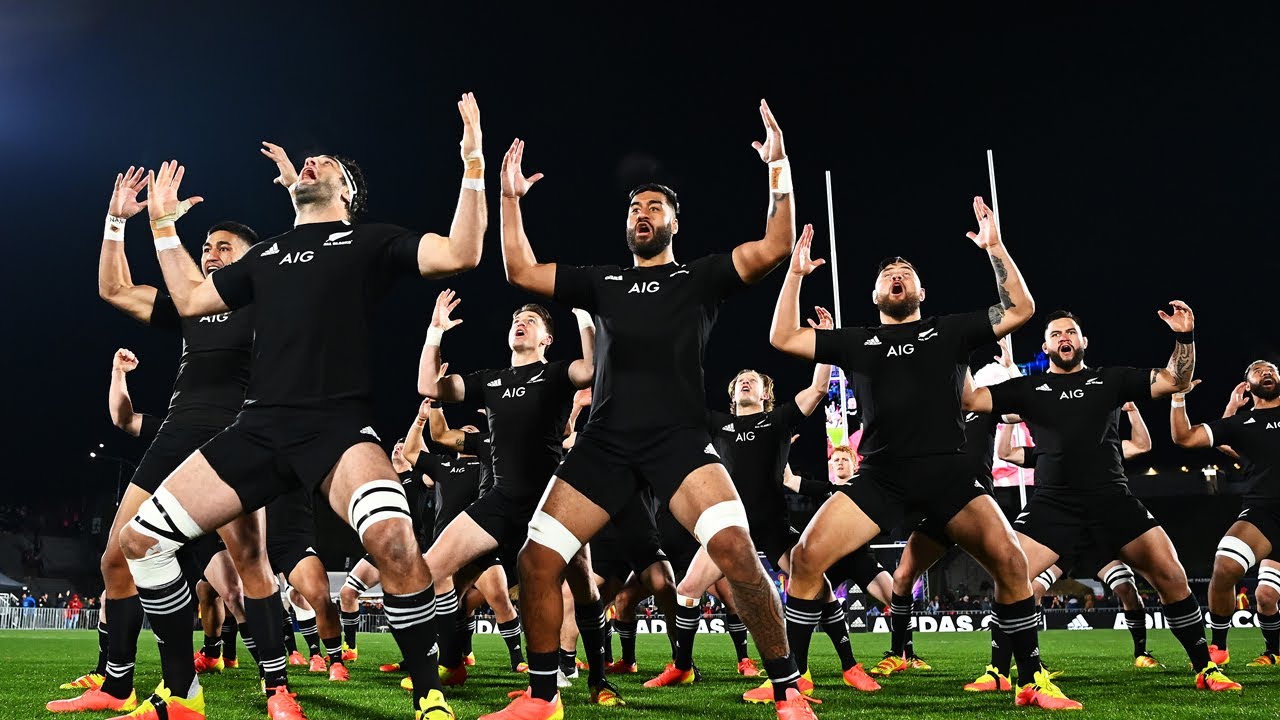The image depicts a team of muscular athletes, likely rugby players, assembled on a green AstroTurf field during a sports event, discernible by the distant spectators and the football goalpost visible in the background. The athletes, all wearing coordinated black short-sleeve sports jerseys and shorts emblazoned with "AIG," are positioned in a triangular formation. They are captured in mid-performance of a synchronized dance: their legs slightly bent, arms outstretched to the sides and up at the elbows, resembling a football goalpost. Additionally, several athletes have white athletic tape around their thighs above the knee. Each athlete is donned in high black socks with three white horizontal stripes at the top and brightly colored neon orange and yellow cleats. Some appear to be shouting, contributing to the dynamic, energetic atmosphere captured under the dark sky.